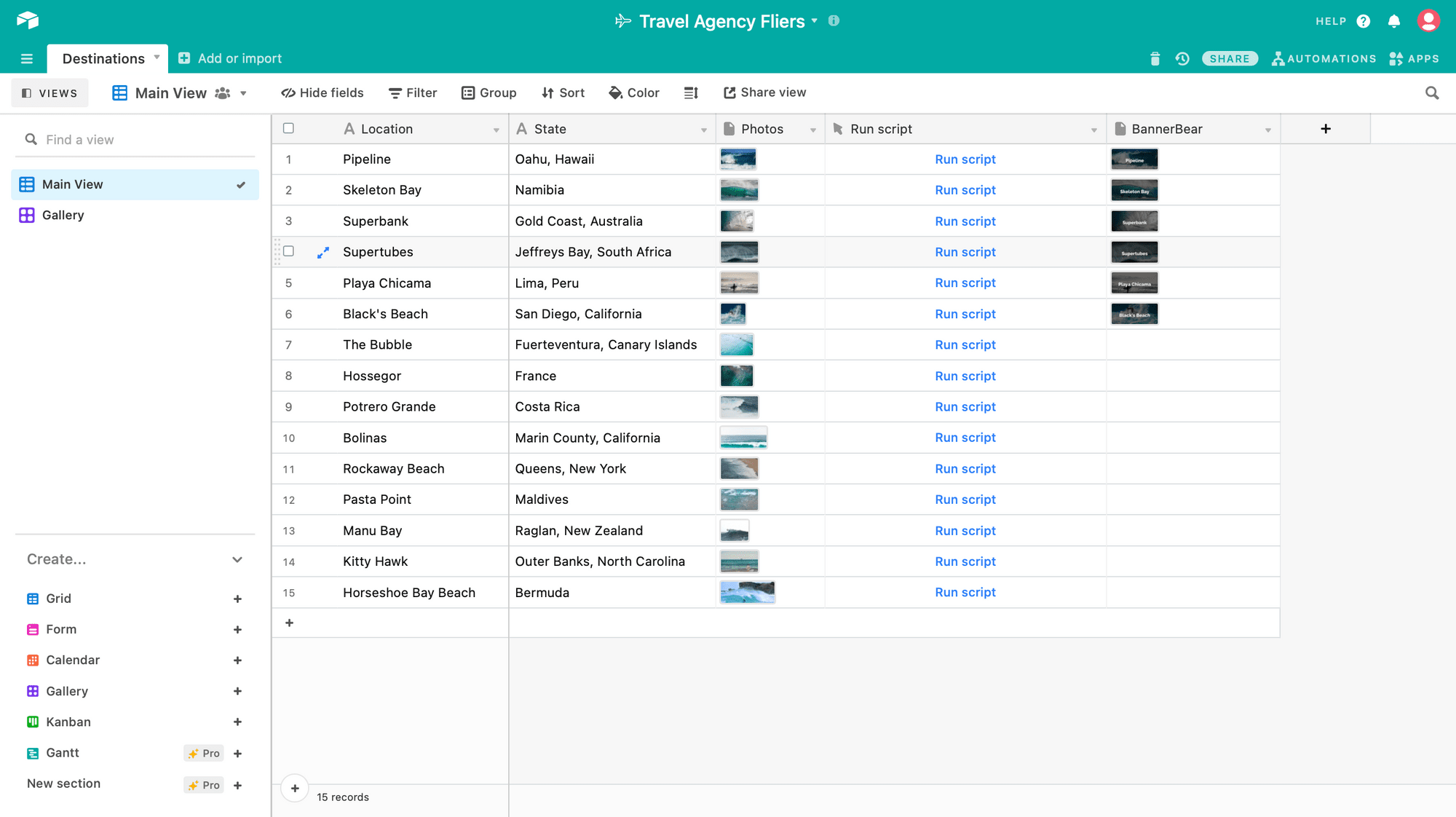In the image, prominently displayed at the top center are the words "Travel Agency Flyers," accompanied by a white airplane icon to their left. On the top right, a set of icons is visible: starting from the right, a pink circular icon with a profile silhouette, followed by a bell icon, and then a blue circle featuring a white question mark. Adjacent to the question mark icon is the word "Help." 

Dominating the middle section of the image is a sequential list of travel destinations, numbered from 1 to 15 and aligned on the left. The entries read from top to bottom as follows: Pipeline, Skeleton Bay, Superback, Supertubes, among others. Corresponding to each destination on the right are the respective states or locations: California, Canary Islands, France, Costa Rica, California, New York, Maldives, New Zealand, North Carolina, and Bordeaux. This detailed layout combines essential travel information with accessible navigation tools and location-specific data.